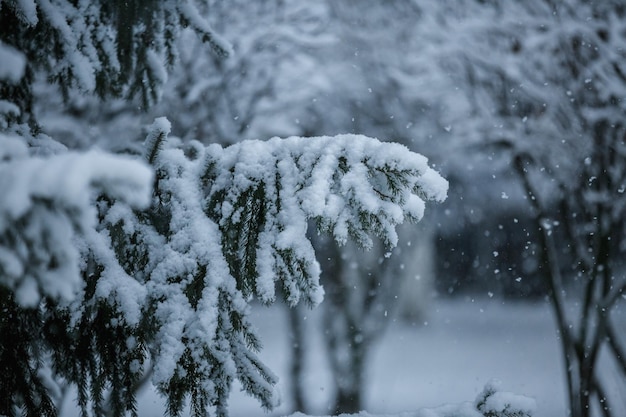This image captures a serene winter scene where snowflakes are frozen mid-air due to the slow camera speed, creating a magical atmosphere. A prominent fir tree branch extends into the frame, heavily laden with about an inch of freshly fallen snow. The snowy branch, possibly from a Christmas tree, is meticulously detailed with long, piney needles visible beneath the snow. Surrounding this main branch, the forest background is a blur of more snow-covered trees, including some with barren branches draped in snow, contributing to the scene's depth and tranquility. The ground is blanketed in snow, and some branches are weighed down so much that they droop towards it, illustrating the heavy snowfall. With no buildings in sight, the focus remains on the natural, snow-coated landscape, encapsulating the peacefulness of a winter forest.